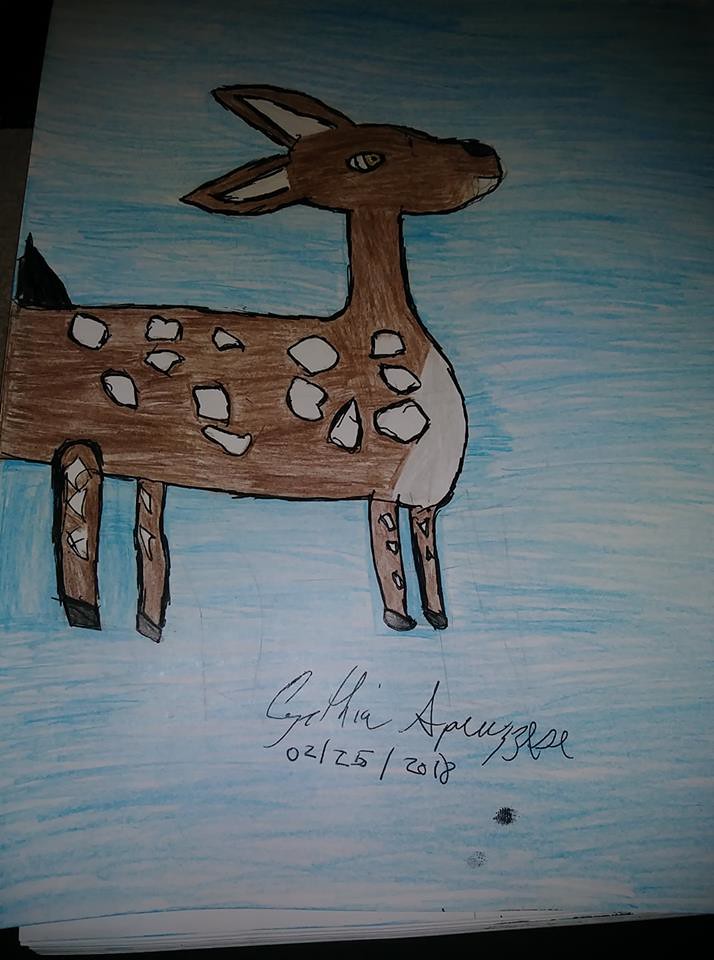This rectangular portrait image showcases a charming drawing, likely by a child, of a deer. The drawing is centered on a vertically-oriented white sheet of paper, which occupies the majority of the image's space. The background includes a slight glimpse of a black surface at the bottom, behind the sheet, and a small triangular slice of a different background in the upper left corner.

The paper itself has been lightly colored with horizontal strokes of light blue crayon, giving the drawing a soft, sketched atmosphere. At the bottom of the page, below the deer, there's a signature written in cursive reading “Cynthia,” followed by an illegible last name beginning with "A" and "P," appearing to be around six or seven letters in total. The date "02/25/2018" is hand-written in black ink below the signature, indicating when the drawing was created.

The deer, positioned above the signature, stretches from the left side towards the center of the image, displaying its right flank. The deer is simply drawn with brown crayon, indicative of a child's work, and features a dozen or so irregular white spots on its side. These spots vary in shape, with some resembling squares and others pyramids. The deer's front chest is marked with a patch of white.

It stands on four straight, thick legs, also brown with a few white spots, ending in black hooves. The tail is depicted as a small black triangle sticking upwards from the rear end. The deer's neck is fairly long and leads to a head that’s an elongated oval. Two pointed ears sit perched atop the head, white on the inside and brown on the outside, facing left. The deer's single visible eye glances upward towards the right corner of the image, while its nose juts out in front.